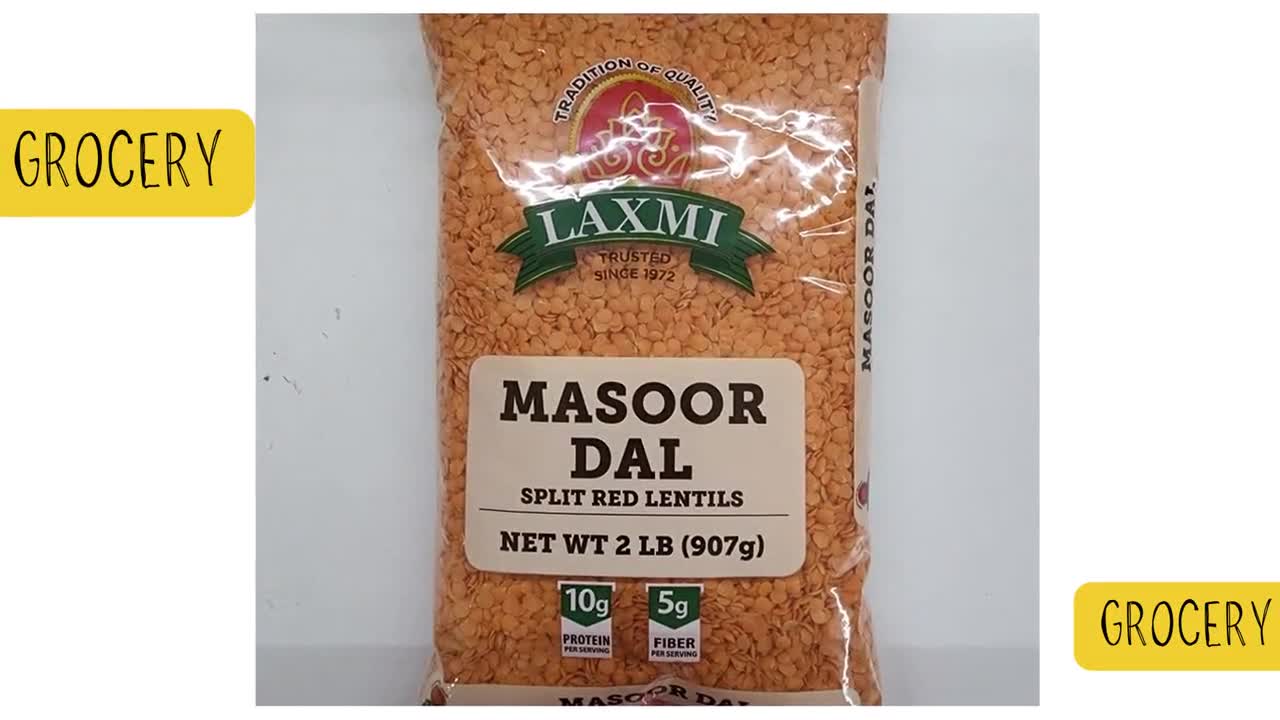The image depicts a large, clear plastic bag of split red lentils propped up against a white wall with some dirt visible on the left side. The bag prominently features the brand name "Laxmi" in white text on a green banner, accompanied by a red and gold logo above it and the words "Tradition of Quality" in a red seal. Right below, "Trusted Since 1972" is written in black text. The label also displays "Masoor Dal" in a white rounded rectangle, followed by "Split Red Lentils" and the net weight "2 pounds (907 grams)." Nutritional information at the bottom highlights 10 grams of protein and 5 grams of fiber per serving. The lentils inside the bag appear orange in color. Additionally, the word "Grocery" is found in black text on a yellow rounded rectangle both at the top left and bottom right corners of the bag. The overall background of the photo is simple, focusing on the product.